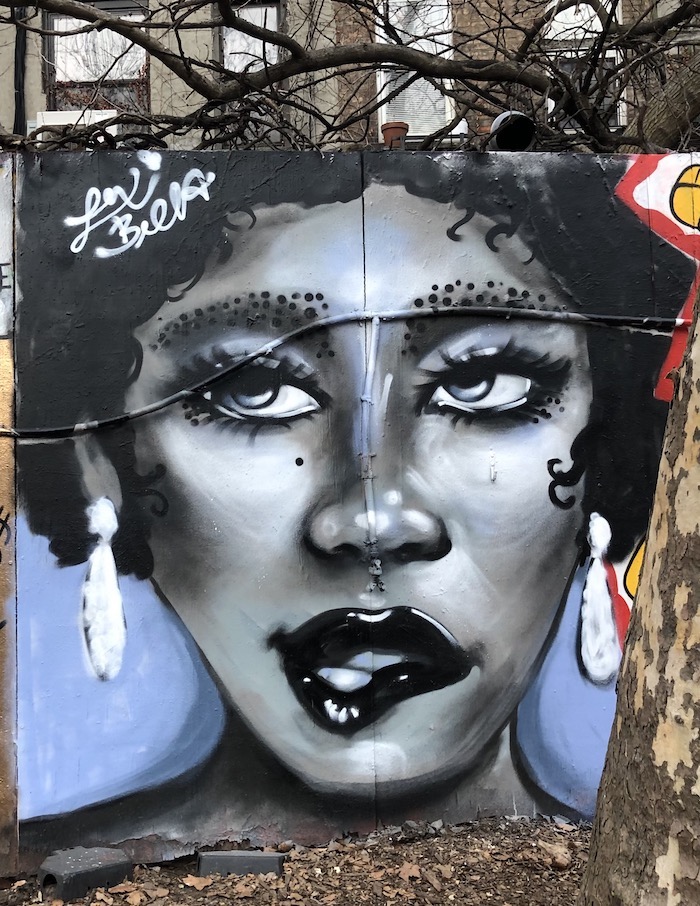In the foreground of this picture, there is a patch of dirt with some scattered leaves, leading to the right where a tree with peeling bark partially enters the frame. Behind this, a wall adorned with graffiti becomes the primary focus. The graffiti is a striking portrait of an African American woman with grayish-blue skin, black lips, blue eyes, and an afro hairstyle. Her expression conveys slight agitation as she bites her lower lip, revealing a touch of white. Her eyebrows are composed of black dots, and she sports long silver earrings. The background of the portrait is painted blue, and there is a pole-like structure running through the artwork. Above the painting, on the upper left-hand side, the artist's signature, likely "Lex Bella," is visible. The upper right-hand section of the wall features a splash of red with white and yellow elements, partially obscured. A potted plant, tree branches, and glimpses of an apartment building with windows add depth and complexity to the backdrop.